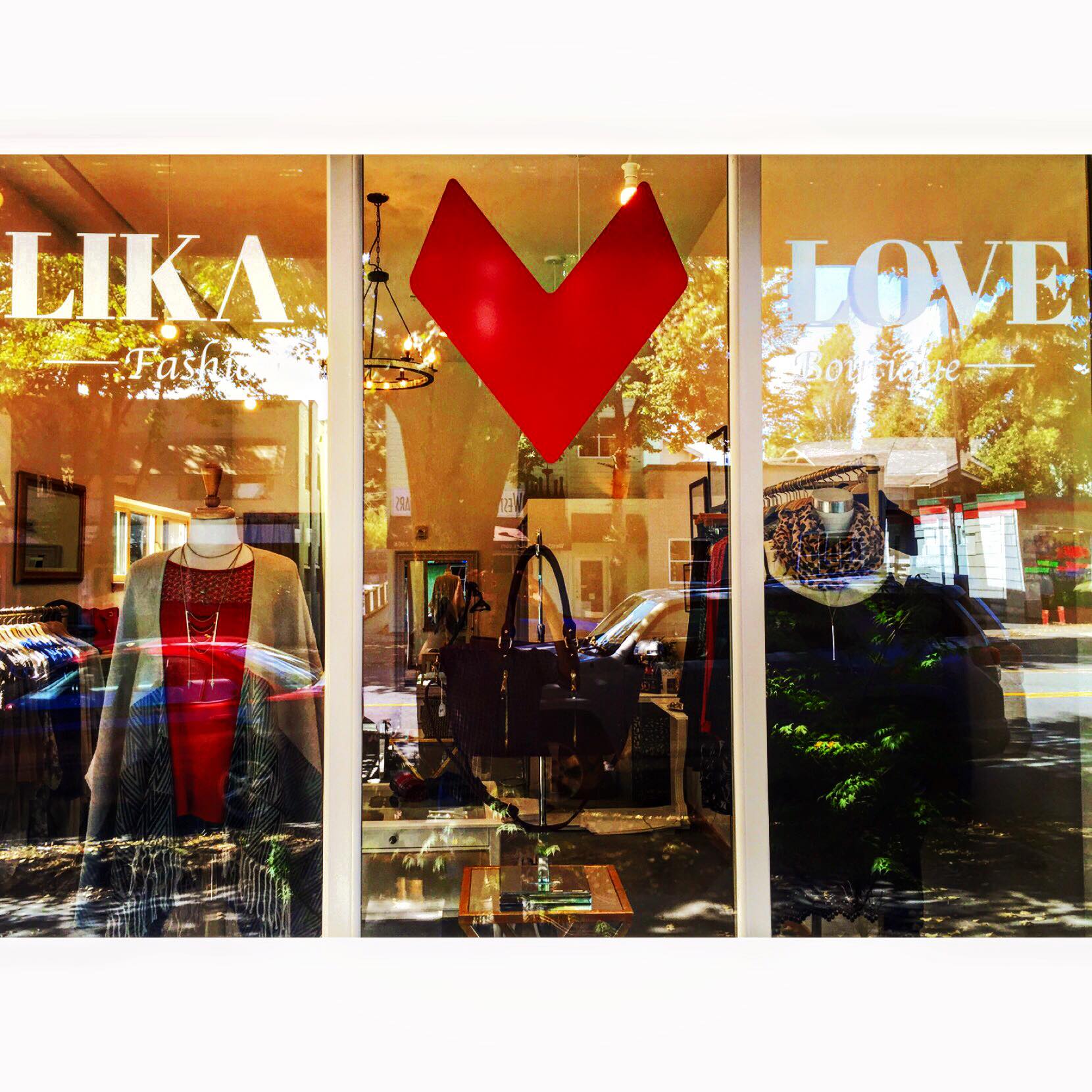The photograph captures the exterior of an upscale fashion boutique, possibly located in a major city like New York or Chicago. The store's name, "Laika Love Fashion," is prominently displayed on the window, which also features a red V, likely representing an abstract heart. The window display showcases various expensive clothing items, such as scarves, jackets, shirts, a sweater with a cardigan, and a necklace. A large black handbag is also visible in the middle of the display. A multitude of colors, especially red, white, and darker shades, dominate the scene. Due to the reflective glass, the image includes reflections of nearby street elements, such as trees, making it slightly challenging to discern all items clearly. The photo is taken from the perspective of someone standing on the street, looking into the boutique.